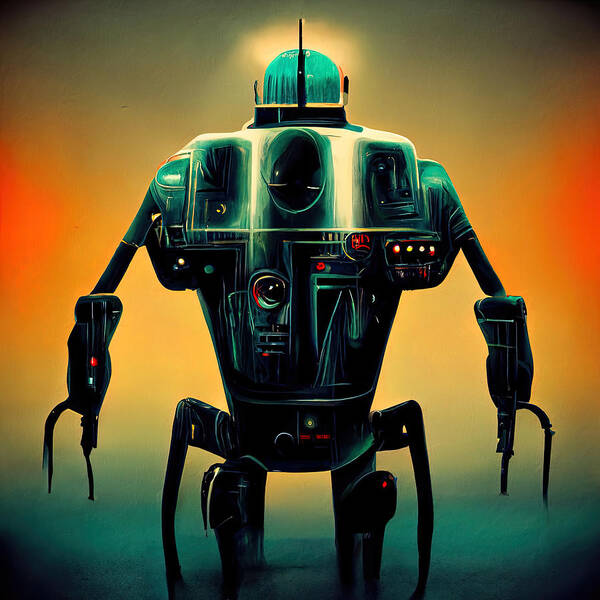This detailed painting features a prominent robot with an intriguing design, set against a striking backdrop. The background transitions from a top band of blackish-gray to a vibrant red with yellow in the middle, and finally settles into a blue area reminiscent of fog at the bottom third of the image. The robot itself is centered and is predominantly blue, white, and black, with a wide, gray body. Its dome-shaped head is teal with a distinctive black stripe running down the side, and it is crowned with a pointy stick resembling a mohawk.

The robot's body is equipped with three dark squares on the front, possibly serving as vents or screens, surrounded by various buttons. At its core, there is a notable black circular feature resembling an eyeball or a camera lens. Its arms are thin at the biceps but culminate in larger hands, each adorned with three sharp, knife-like extensions. Additionally, gadgets can be seen on the robot's wrists, adding to its intricate design.

The robot's waist features a thin strip with small red writing below it. It stands on four legs: two robust legs extending straight down and two more that branch off from the hips horizontally before thinning and descending like spider legs. The robot's appearance evokes a crab-like quality, with claws for hands and legs. Its entire form is slightly illuminated by the gradient orange-blue background, highlighting its futuristic and mechanical complexity.